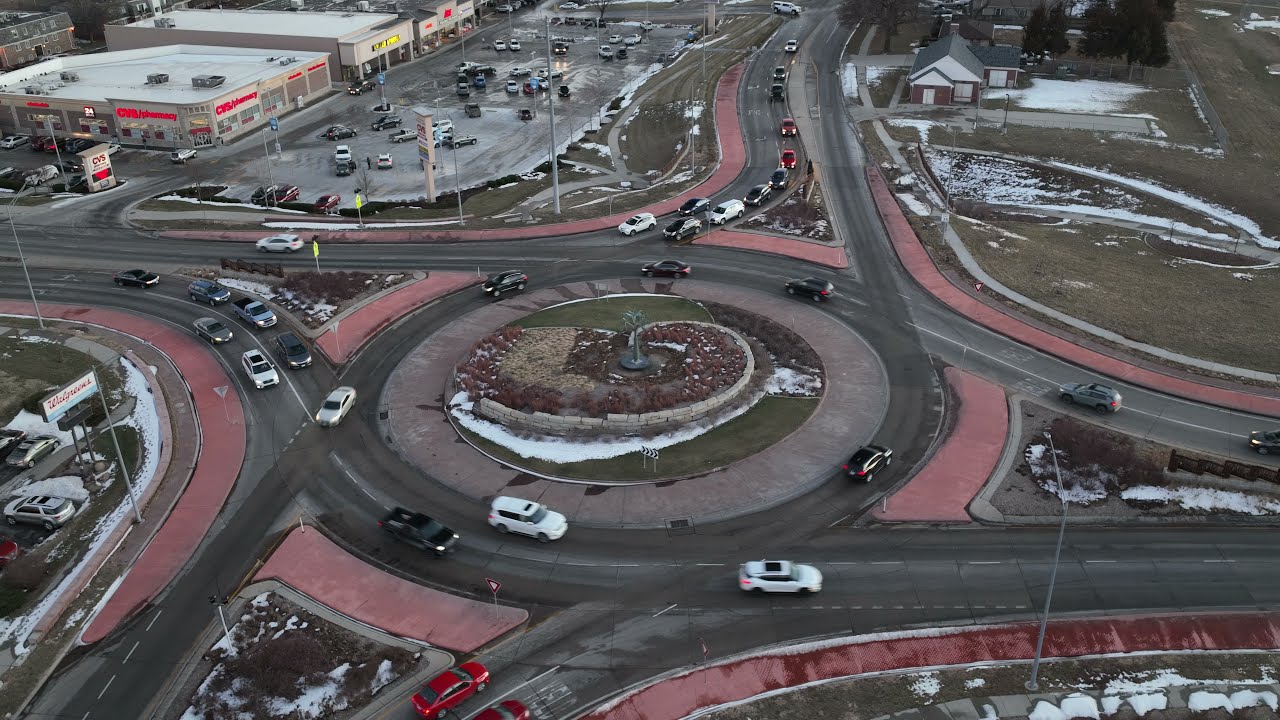The image captures a clear, overhead view of a bustling cityscape centered around a roundabout. Dominating the center, the roundabout features a steel monument resembling a tree encircled by a spiral of bricks. Roads branch out from the roundabout in various directions, specifically extending towards the top, left, right, and bottom of the image. Traffic moves in a counterclockwise pattern around the roundabout, with several cars navigating both towards and around it. Surrounding the roundabout are various buildings and parking lots, including a recognizable CVS Pharmacy located in the top left corner and an Ace Hardware store positioned towards the top center. The scene is depicted in full color, showcasing a palette of red, black, white, gray, maroon, and brown. Snow is visible on the ground and on the roundabout, indicating a snowy setting. The image appears to be taken during daylight hours, with ample natural light illuminating the scene. The overall layout appears somewhat scattered, giving a comprehensive view of the diverse elements within this urban landscape taken from an aerial perspective.